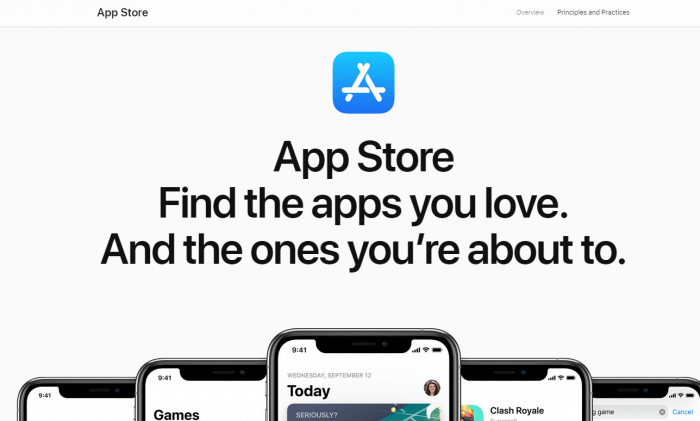The advertisement showcases the App Store with the word "App Store" prominently displayed in the top left corner, accompanied by "Overview and Principles and Practices" on the right. Below these headings is a gray box containing a blue square background with a stylized 'A' made from popsicle sticks. Beneath this, in bold black text, are the words "App Store: Find the apps you love and the ones you're about to."

Central to the image are five staggered iPhones. The three on the left display the time as 9:41. In the forefront, an iPhone showcases a screen titled "Wednesday, September 12" with the word "Seriously?" and a woman's avatar in the top right corner. The following iPhone screen features the game "Clash Royale." The remaining two iPhones on the right also show Wi-Fi connectivity with four bars and fully charged batteries. The backmost iPhone screen includes a visible "Cancel" button and a search bar on the right, while the back left screen is blank except for the time.